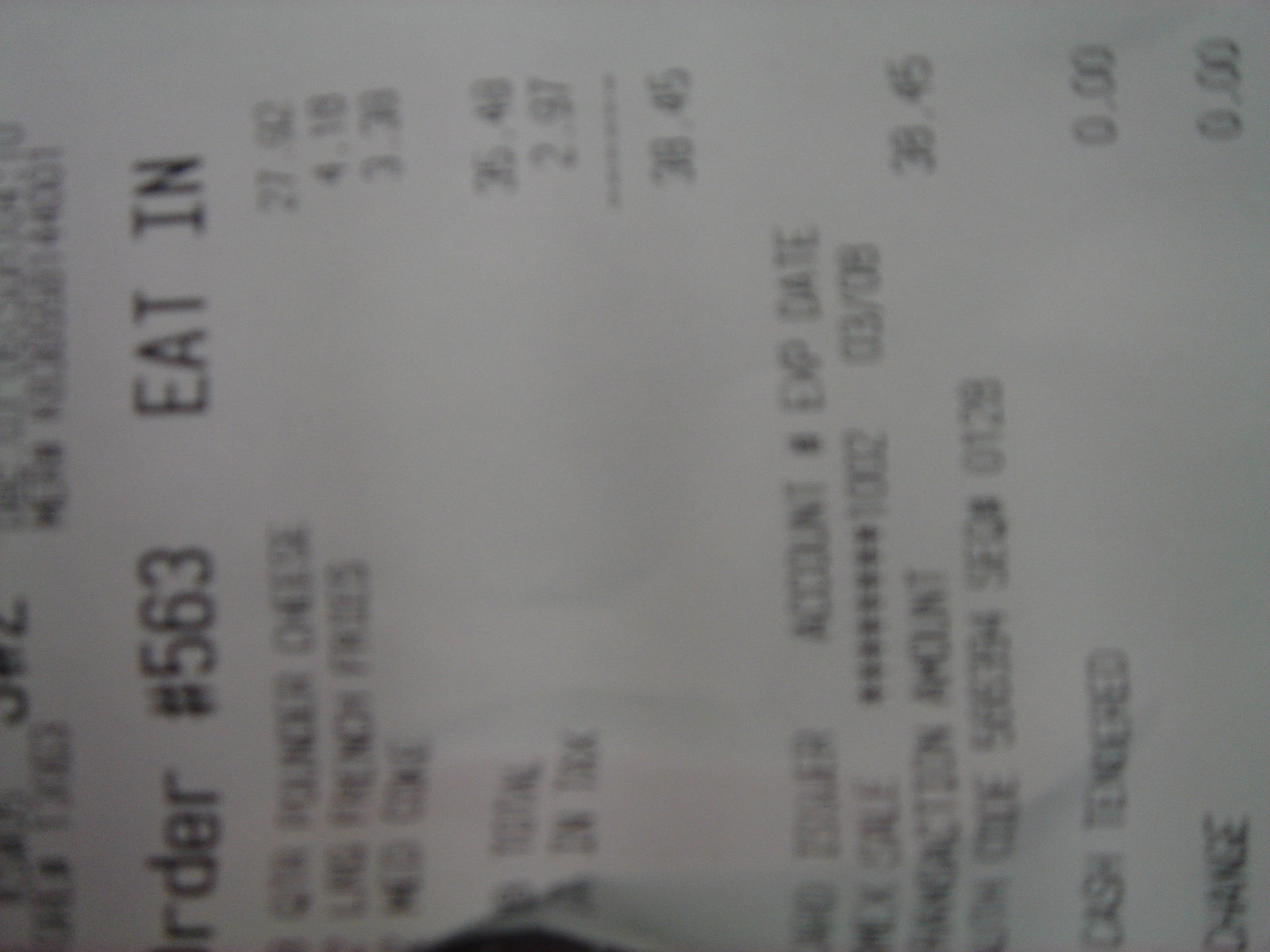This is a very close-up and out-of-focus photograph of a receipt, positioned sideways in a horizontal fashion, making the text appear vertical from left to right. The receipt is primarily white, albeit a light gray due to the shadow and blurriness, with all text in black. The most legible portion along the left side of the image reads, "Order number 563, EAT IN." Beneath this, although partially obscured, are itemized listings that include "cheese," "large French fries," and "medium Coke," with respective prices of 2792, 418, and 338. The tax amount reads 297 and the total is stated as 3845. The receipt also indicates that no tip was given and there were zero changes. Some credit card details are also mentioned but remain illegible due to the blur. There is a small section where the receipt is wrinkled and folded, adding to the obscurity of some of the text.